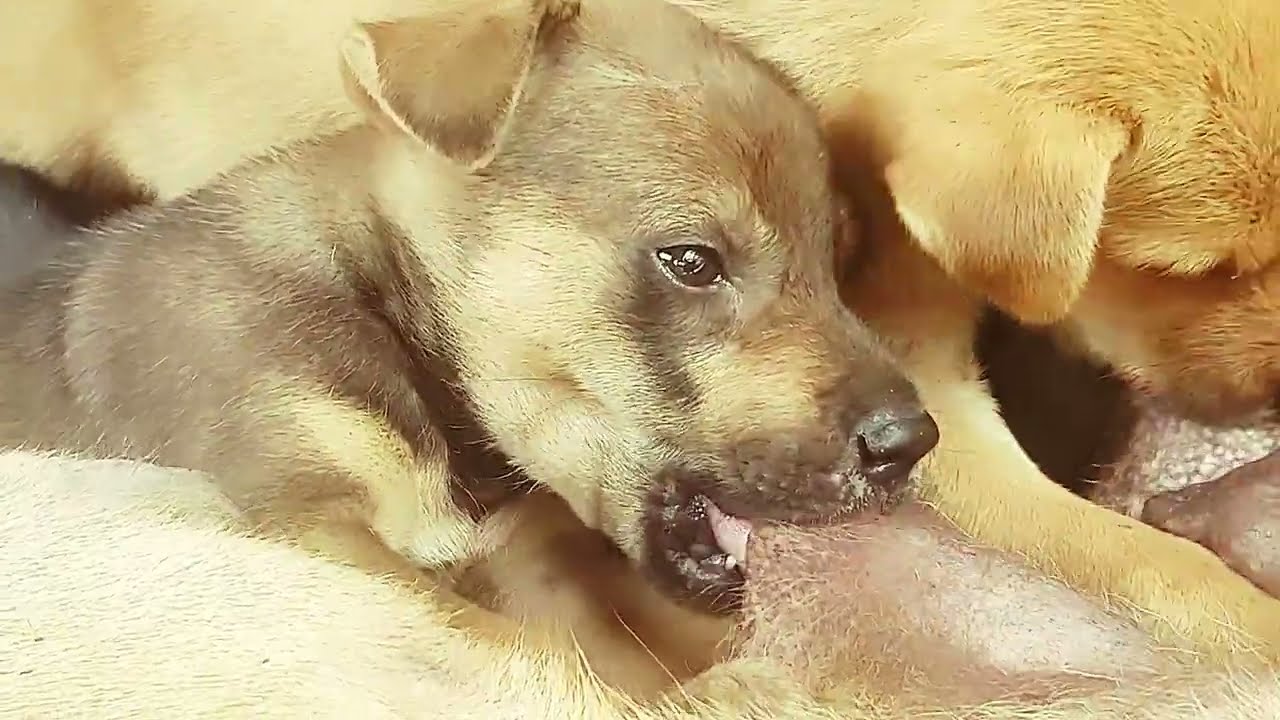This vibrant color photograph captures an intimate close-up of two puppies nestled together on a cream-colored floor. The focal point is a small brown and white puppy with shiny brown eyes, a black nose, and a brown muzzle. This puppy has a bit of black around his lips and one visible floppy ear. This adorable pup appears to be nibbling on the body part of another puppy beside him, though it is unclear if he is gnawing on a leg, a tail, or some other object. The second puppy is only partially visible with fur ranging in golden brown and reddish hues and presenting one floppy ear as well. They both sport short-haired coats and exude a playful energy, suggesting they were caught in the midst of a playful moment. The natural lighting accentuates their expressive features and the warmth of their fur, adding to the charm of this detailed and engaging scene.